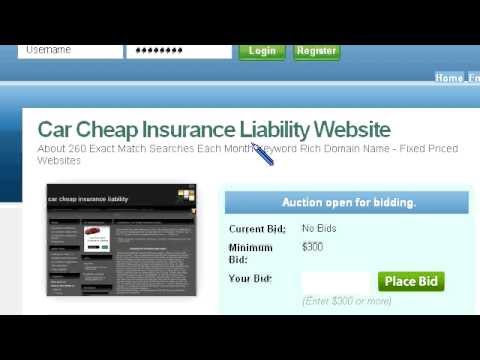The image showcases a login page for a website with a split-color background—blue on the top half and white on the bottom half. On the top left side, there is a text box for entering the username, followed by a password text box to its right, which displays the password as black dots. Further to the right of the password text box are two green buttons labeled "Login" and "Register," respectively.

At the bottom portion of the image, green text reads, "Car Cheap Insurance Liability Website," followed by additional descriptive text: "About 260 exact match searches each month. Keyword-rich domain name. Fixed price."

On the far right side of this section, there is a notification stating, "Auction Open for Bidding," with "Current Bid: No Bid" and a minimum bid requirement noted as "$300." Below this, there's a field labeled "Your Bid" where users can enter their bid amount with a prompt to "Enter $300 or more." To the right of this field is a green button with white text reading "Place Bid."

On the left side of this bottom section, there is a sample webpage display. This sample is displayed with a black background and features the text "Car Cheap Insurance Liability" in white. The overall impression of the sample webpage is one of a simplified or perhaps even a placeholder design, given its minimalistic presentation.